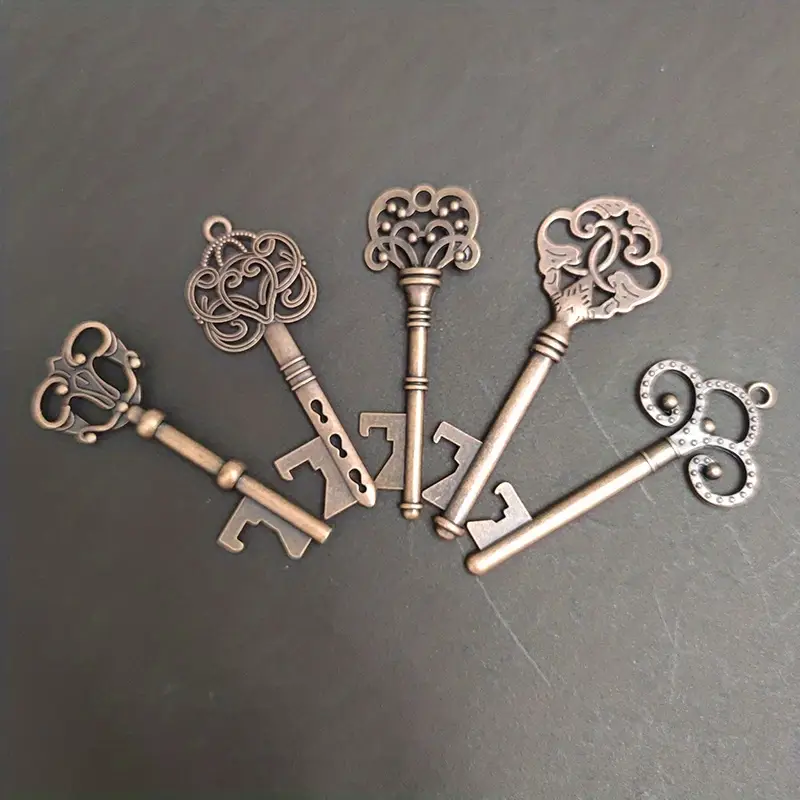The square, full-color photograph, taken indoors using artificial lighting, features a collection of five old-fashioned skeleton keys, meticulously arranged in a fanned-out, half-circle shape. The background is a textured gray surface, with noticeable scratch marks where the keys have contacted it, and it brightens considerably in the lower right-hand corner due to the artificial light source. The keys exhibit an ornate and elaborate design, made from brass, showcasing a bronze-like finish with intricate details. Each key has a long shaft leading down to unique and decorative handles at the top. These handles vary in design, featuring intricate curves, interlaced loops, beaded accents, and even heart-like shapes. The keys lie against the dark gray background, creating a visually striking contrast with their dark brass color.